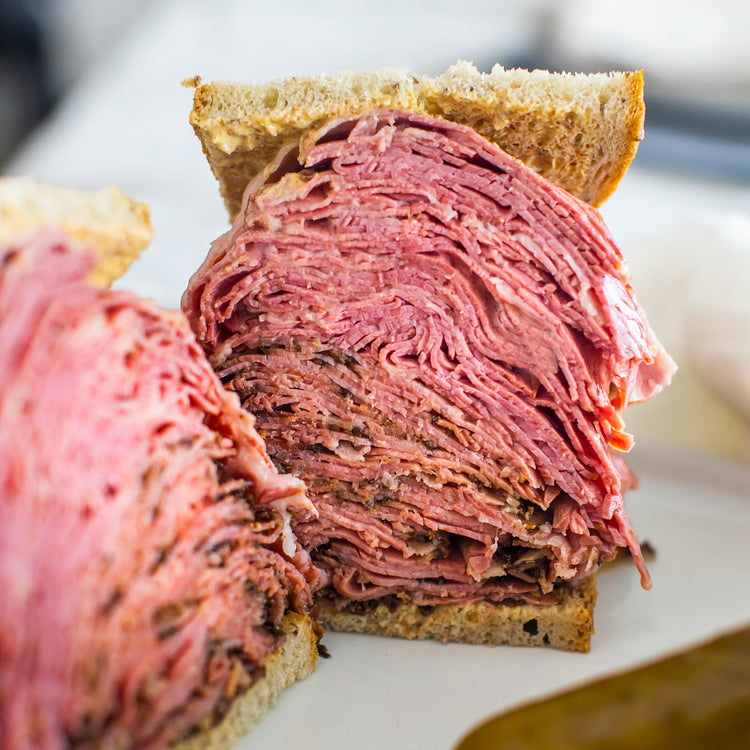The photograph features an enormous sandwich sitting on a white surface, potentially butcher paper, placed on a brown, wooden table. The sandwich, made from whole wheat bread, has been sliced in half and separated to reveal its contents. Each half showcases an impressive, towering pile of thinly sliced meat, with ham filling the top half and roast beef in the bottom half. The background is blurry, putting the focus on the thick, dense layers of meat and the delicate slices of bread. Despite being thin, each slice of bread nearly disappears beneath the substantial mound of meat in the center. The bread appears to have a spread of mustard or butter on the underside, contributing to the overall texture and flavor of the sandwich.